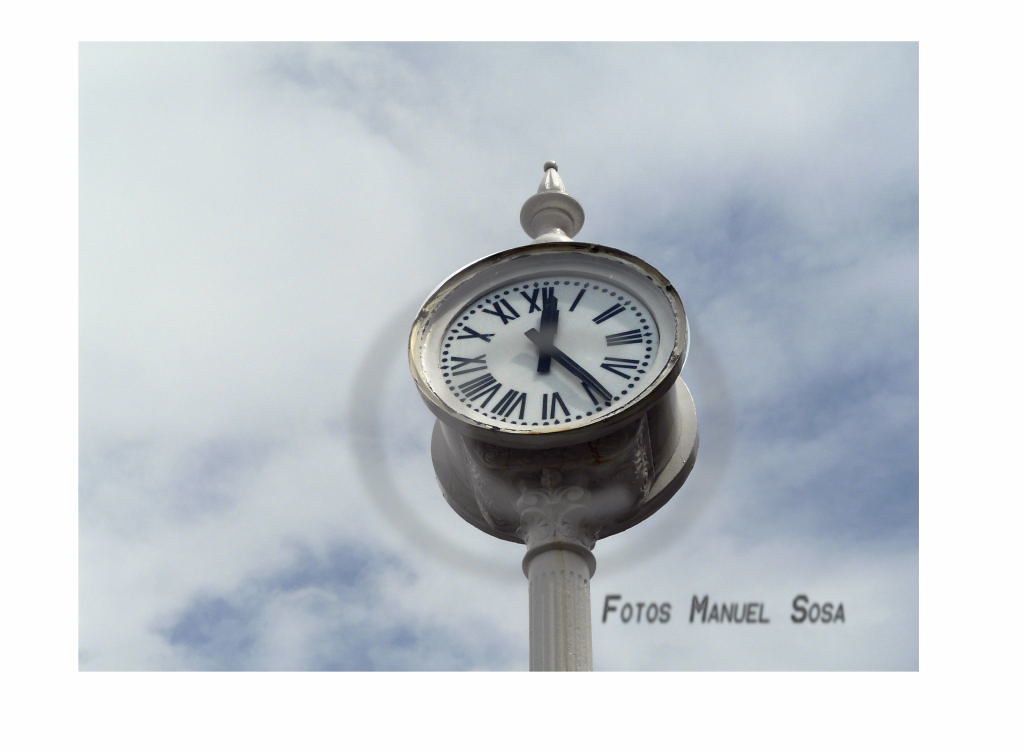The photo, taken during the day, features an old-fashioned clock with black Roman numerals and hands, prominently displaying the time 12:25. The clock is mounted on a tall, white ribbed post that culminates in a pointed finial at the top. The clock has a dual-faced design, with the visible face framed by a dark pewter-colored rim, which adds a touch of contrast against the predominantly white structure. The backdrop includes a sky that is mostly covered with white clouds, with hints of blue peeking through, creating a soft, overcast ambiance. The photograph bears the signature "Photos Manuel Sosa" in the lower right corner, attributing the artistic credit to the photographer. The entire arrangement exudes a quaint, vintage charm, accentuated by the detailed craftsmanship of the clock and its mount.